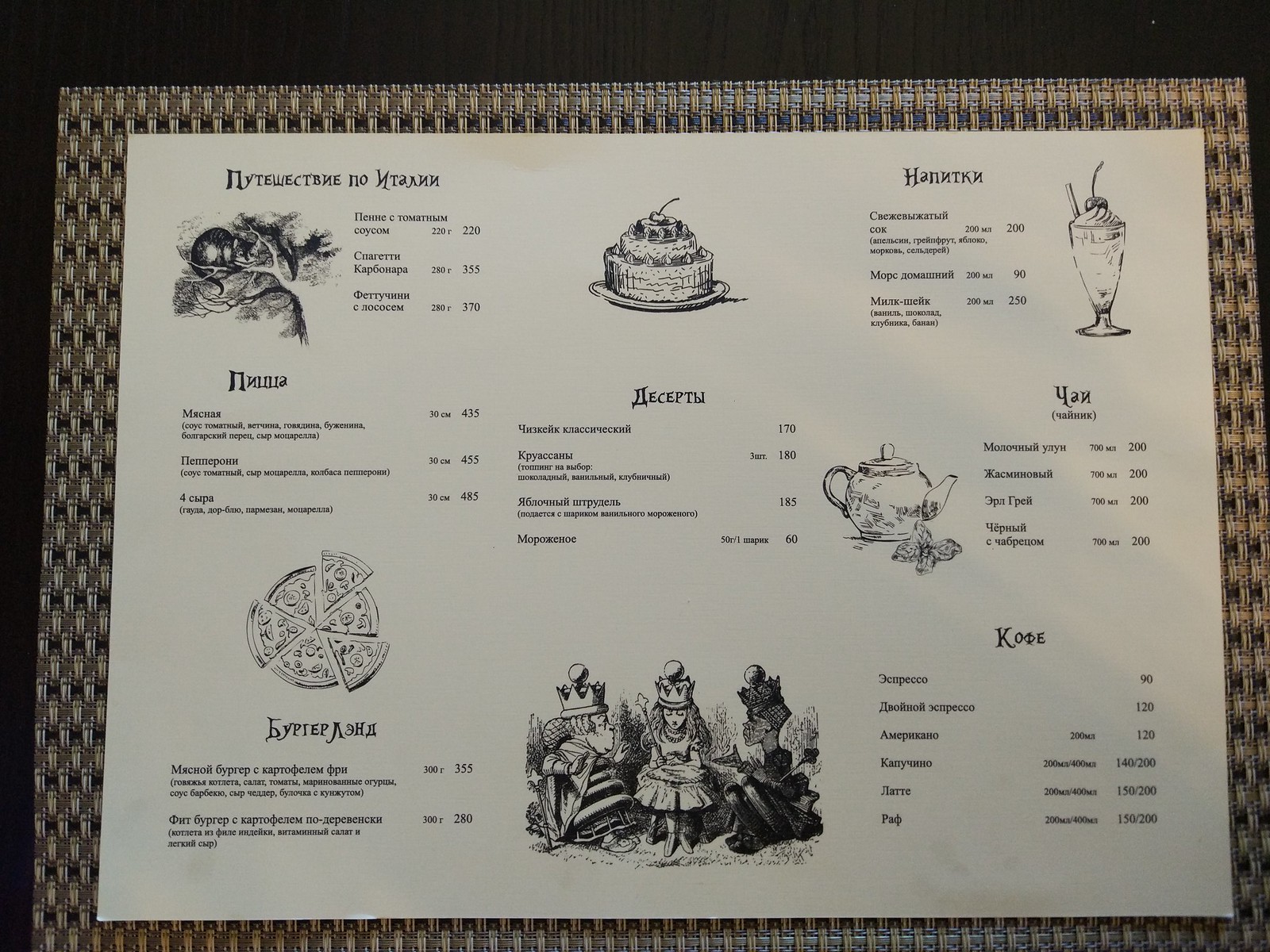A detailed photo of a menu printed in Russian, featuring designated sections with accompanying images for various food items and beverages. The menu is meticulously presented on tan paper with white ink, resting on a rattan-like placemat or table surface. It is structured into three distinct columns:

- The left-hand column comprises three sections, with an image of a pizza at the top and an indiscernible graphic further down.
- The middle column is divided into two sections, showcasing an image of a cake at the top, followed by an illustration of three small figures wearing crowns beneath it.
- The right-hand column also consists of three sections, starting with an image of a milkshake, and directly below it, a teapot.

Each section lists menu items alongside corresponding prices, although the text is in Russian and not readable. The ambient lighting appears to be coming from the right side, casting soft shadows that highlight slight wrinkles in the menu paper, adding depth and texture to the overall presentation.